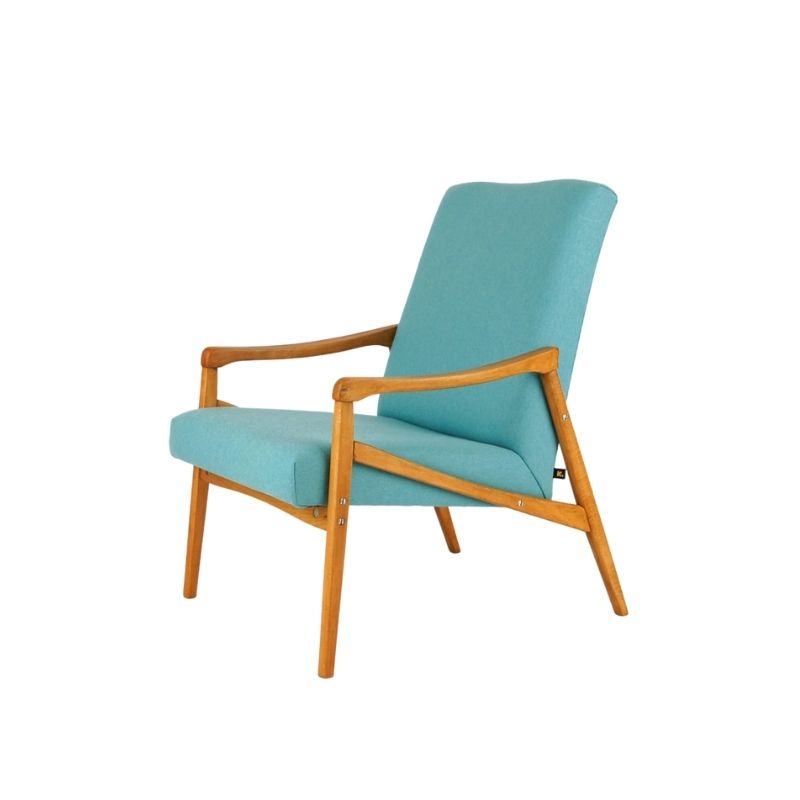This image depicts a teal-colored lounge chair, evoking a mid-century modern aesthetic, possibly with a hint of vintage flair. The chair features a light brown, wood-stained frame, securely held together with screws, showcasing its sturdy construction. The frame includes four slightly flared legs, diagonally supported for added stability, with the armrests subtly curving downwards. The teal upholstery covers both the seat and the tall back, giving it a refined look. A small black rectangular tag with white writing, possibly a logo, is visible on the upper back of the chair. The detailed presentation and the white background suggest that this is a product image, similar to those found on shopping sites like Amazon, highlighting the chair's elegant and timeless design.